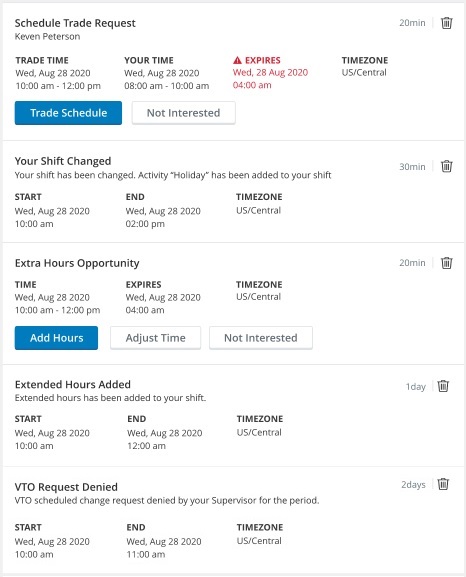Certainly! Here is a more polished and detailed version of the provided caption:

---

The image features a clean layout with a white background, divided into five distinct rows by thin, light gray lines. These lines are subtly placed between each row, enhancing the organizational structure. 

1. **First Row - Schedule Trade Request:**
   - At the top left, bold black text reads "Schedule Trade Request".
   - Below, in smaller text, the name "Kevin Peterson" is displayed.
   - The row is divided into four columns, each with text in all caps:
     - **TRADE TIME:** A long horizontal blue rectangle containing white text, "Trade Schedule".
     - **YOUR TIME:** Adjacent to the right.
     - **EXPIRES:** Red text positioned further right.
     - **TIME ZONE:** More black text aligned to the far right.

2. **Second Row - Your Shift Changed:**
   - Prominent black text states, "Your Shift Changed".
   - Below, a descriptive line reads, "Your shift has been changed. Activity holiday has been added to your shift."
   - This row features three columns:
     - **START:** Start time details.
     - **END:** End time details.
     - **TIME ZONE:** Relevant time zone information.

3. **Third Row - Extra Hours Opportunity:**
   - Centrally positioned, bold black text announces, "Extra Hours Opportunity".
   - Underneath, the following three columns are listed:
     - **TIME:** Scheduled time.
     - **EXPIRES:** Expiry details.
     - **TIME ZONE:** Specified time zone.
   - Following the columns, a rectangular blue box with white text states, "Add Hours". To its right, two smaller white boxes with gray outlines read, "Adjust Time" and "Not Interested".

4. **Fourth Row - Extended Hours Added:**
   - Black text indicates, "Extended Hours Added".
   - Below, a note specifies, "Extended hours have been added to your shift".
   - Similar to previous rows, it contains three columns:
     - **START:** Start time information.
     - **END:** End time information.
     - **TIME ZONE:** Corresponding time zone.

5. **Fifth Row - VTO Request Denied:**
   - Bold black text at the bottom reads, "VTO Request Denied".
   - Below, it explains in smaller text, "VTO schedule change request denied by your supervisor for the period."
   - The row is split into three columns as well:
     - **START:** Start time details.
     - **END:** End time details.
     - **TIME ZONE:** Relevant time zone information.

---

This descriptive caption thoroughly details the image's layout, ensuring clarity and focus on the distinct features within each row.